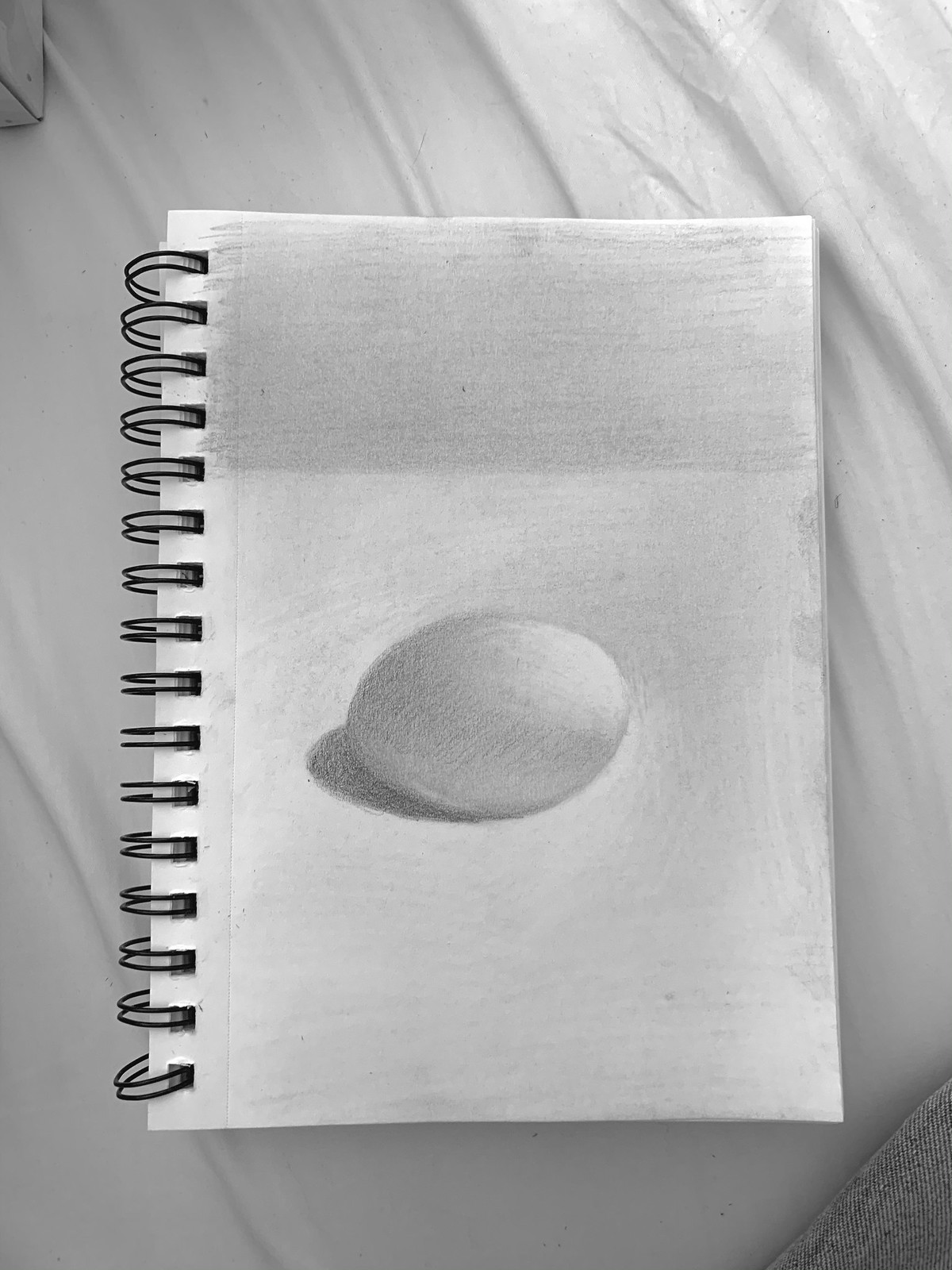The image displays a small sketchbook featuring a black spiral spine and perforated pages. Resting on a white sheet with a corner of gray, wrinkled fabric peeking in from the bottom right, the sketchbook's top page showcases a detailed, pencil-drawn egg. The egg, positioned on its side, is lightly shaded and appears three-dimensional against a predominantly gray background. This shading gradually transitions from darker at the top to lighter at the bottom. The egg's left side casts a perfect, darker shadow, enhancing its realistic, rounded contours and giving it a lifelike presence on the paper. The meticulous use of shading and shadows accentuates the egg's curvature, creating a striking, almost tangible visual effect.